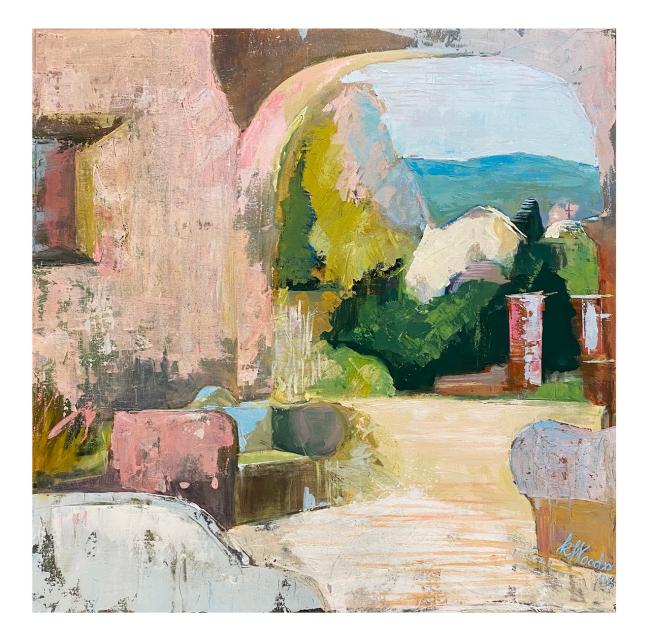The painting depicts an outdoor scene as seen from a porch, framed by an archway. On the left side of the canvas, there's an old building with peeling pink paint, revealing patchy green areas underneath. A window with a wooden frame, featuring a light brown vertical line and a light red inner line with blue blotches inside, sits on the left edge of the building. Below the window, the ground is adorned with square elements, including one brown square splattered with pink paint, and another, in the bottom corner, resembling the front of a car with a sloping, flattened shape.

Attached to the left side of the building is an archway with intricate details: a brown spot on top, and pink and yellow paint on the inside, marred by a gray patch where the paint is peeling. Through the archway, the backdrop reveals distant mountains in light blue and teal hues, with painted green bushes—some shaded darker with lighter green highlights on top. To the right, two cylindrical structures stand upright, one painted in brown and pink, and the other mainly in white and light pink. Another cylinder, connected to the side of the archway, features a brown background striped with white and is tethered to the archway by white lines.

The scene extends into a light peach-colored clearing to the right of the building, enhancing the spacious open-air ambiance. The sky above and the hills in the backdrop are bright and vibrant, with the natural lighting illuminating the vivid colors of the scene. In the bottom-right corner, a signature in blue ink reads "K MOODA," adding a personal touch to the artwork. This painting, possibly created with watercolor or oil, combines a rich palette of colors like white, light blue, green, yellow, red, brown, and pink to bring this serene outdoor setting to life.